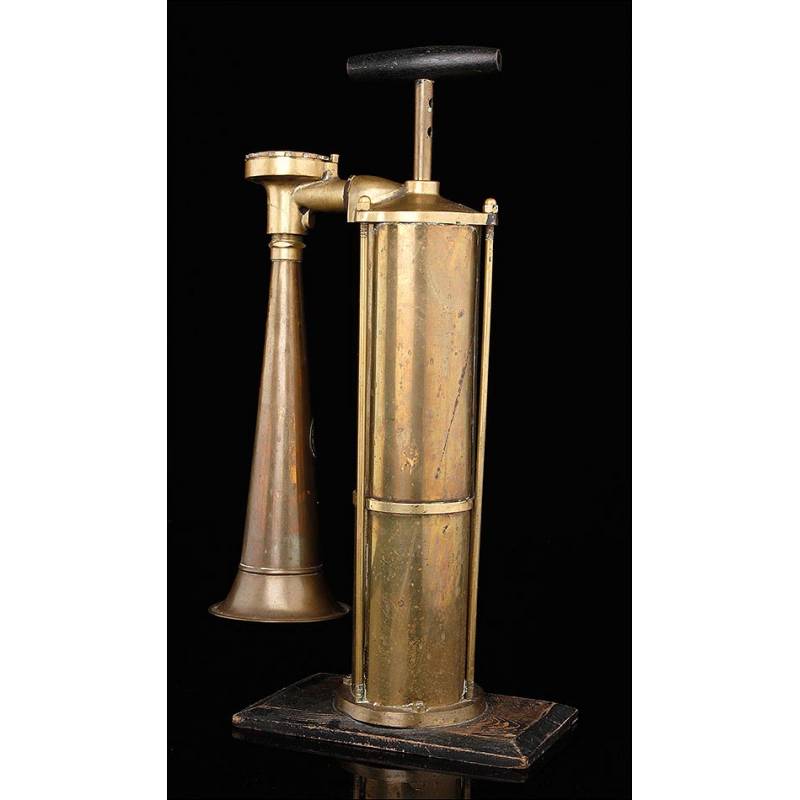The image depicts a sculpture or mechanism set against a pitch-black background, drawing complete focus to the object. The centerpiece is a large, golden-bronze cylinder prominently standing vertically. This main cylindrical structure is supported by several thinner rods and features a central gold strap around its midsection. At its base, the cylinder rests on a shiny, brown-bronze plate, which also reflects the mechanism. At the top of the main cylinder, there is a plunger-like component, resembling an old-fashioned dynamite pump or bike pump with a wood-like handle. Adjacent to this, a horn-like structure curves out to the side, becoming wider towards its mouth, suggesting it might function as an old-fashioned horn. This intricate blend of metals and designs evokes a sense of antiquity and mechanical artistry.